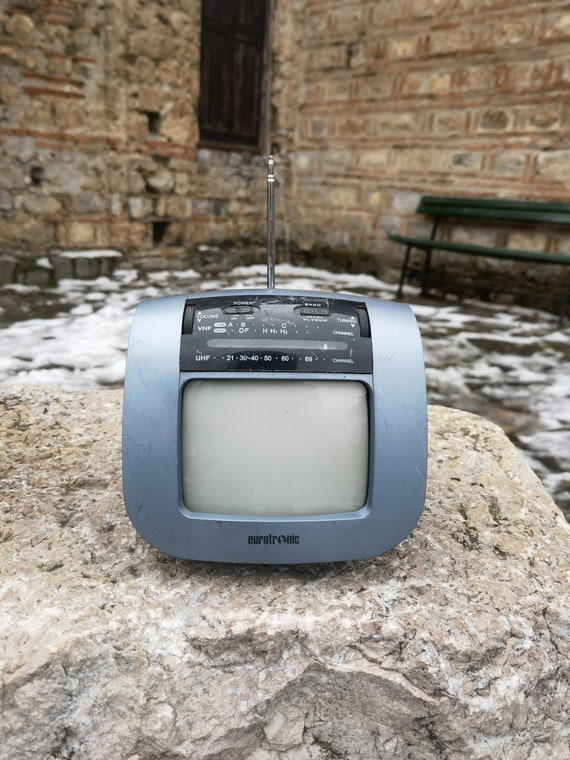The photograph captures an old-fashioned radio-television combination device, characterized by a square, rounded-edge design with a steely blue or gray plastic casing. The top portion of the device features a traditional radio with dials, while the bottom section houses an unlit television screen. A slender, silver antenna extends centrally from the top. The brand "Eurotronic" is printed at the bottom, replacing the letter 'O' with an image of the Earth. This equipment sits atop a gray-tan boulder, situated within a small, walled-in courtyard. The background reveals a green bench to the upper right and tall stone masonry walls, with a snowy, icy sidewalk contributing to the scene's cold, wintry ambiance.